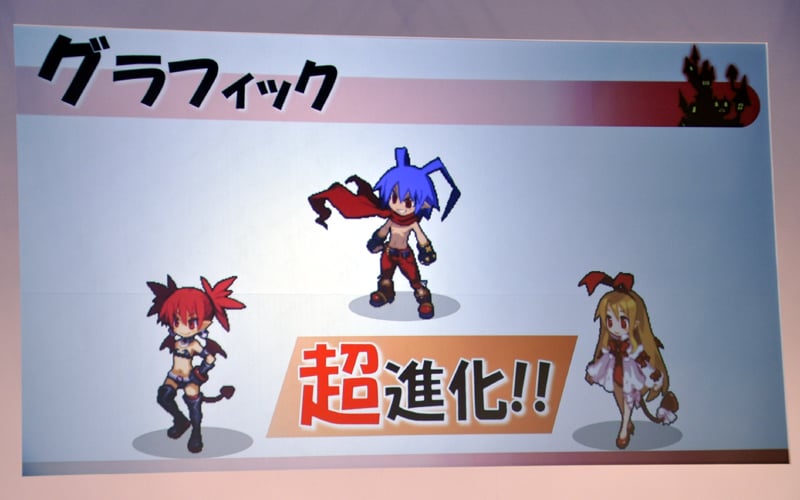A meticulously detailed image features several unique elements. At the top left corner, black text overlays the picture, although the language is Japanese, which I cannot read. On the top right, a whimsical yet haunted cartoonish castle appears, cast in a dark red hue and emanating a red glow that heightens its eerie atmosphere.

The three distinct characters presented in the image each have their own visual flair:

1. On the left, a young demon girl is depicted, scantily clad, with vivid red hair styled into pigtails secured by two small buns on either side of her head. She boasts a mischievous demeanor with a demon tail and thigh-high boots that accentuate her devilish allure.

2. Center stage is a character named Little Heart. He has striking blue hair, with two strands standing out prominently. Little Heart exudes a rugged yet charming look, wearing a scarf around his neck while his torso remains bare. His outfit includes black gloves, red pants, and sturdy Boots, emphasizing his adventurous spirit.

3. On the bottom right, a girl with flowing blonde hair captures attention. She adorns a red band topped with bunny ear-like protrusions, matching her red eyes. Her attire consists of a red and white dress accompanied by red heels, completing her vibrant and playful appearance.

In summary, this richly illustrated image captures a blend of whimsical and eerie elements, highlighted by the striking and diverse characters vividly brought to life within the scene.